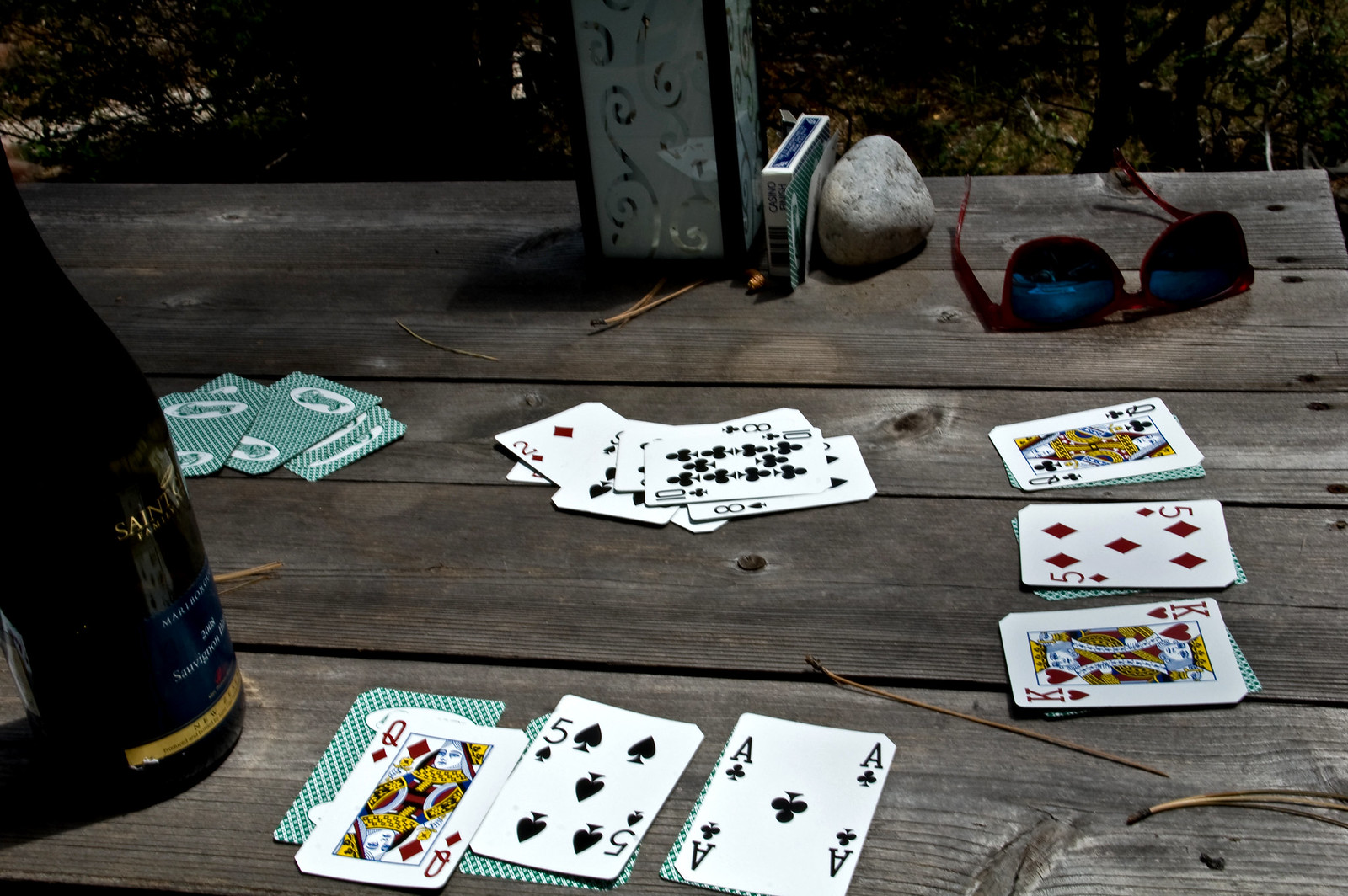This horizontal image captures an intimate scene at an outdoor picnic table, showcasing a lively moment of a card game in progress. The table itself is made of weathered wood, hinting at its long-standing presence under the open sky. Scattered across its surface are playing cards that players have left where they last placed them. In the background, lush trees add a touch of natural serenity to the setting.

Several notable objects rest on the table. A pair of sunglasses lies casually amidst the playing cards, while a weathered rock serves as a makeshift paperweight. The deck of playing cards, still in its case, is turned on its side, seemingly abandoned in the midst of the game. An unlit lantern, with its panes glinting in the sunlight, suggests preparations for extended play into the evening. Additionally, a dark bottle of some beverage sits to the left of the cards, ready to refresh the participants.

In the center of the table, playing cards are arrayed face-up, likely part of an ongoing game. In front of two seats, three neat stacks of cards are visible, with the top card in each stack face-up and the rest face-down underneath. This pattern repeats at the other end of the table, while a lone pile of face-down cards suggests an unorganized hand waiting for a player to take their turn.

The scene is bathed in daylight, with the sun casting gentle shadows and enhancing the inviting atmosphere. The overall impression is one of relaxed enjoyment as friends or family prepare to engage in a friendly game of cards, surrounded by the warm embrace of nature.